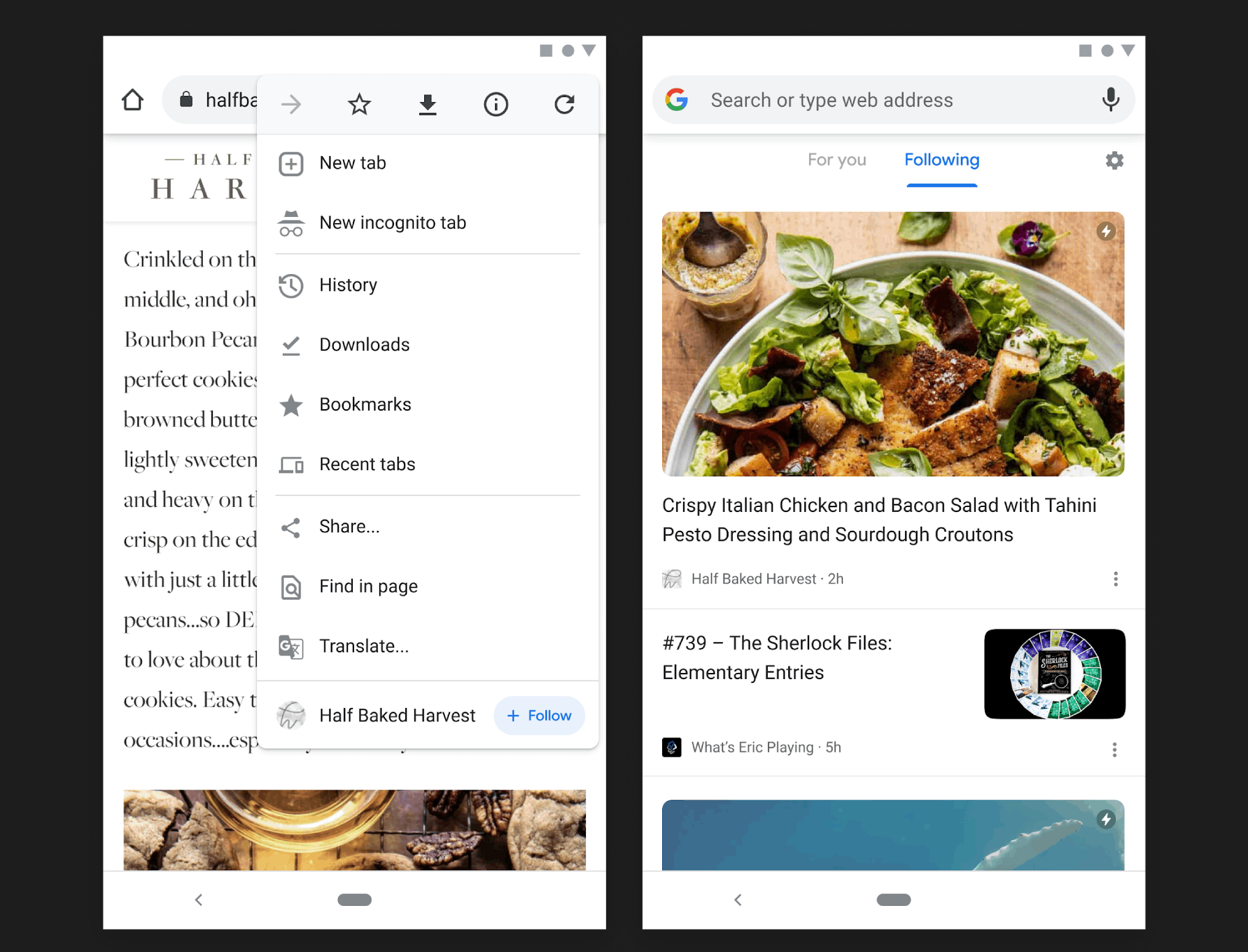A composite screenshot featuring a black background showcases two diverse web elements. On the left, a browser menu includes options such as "New Tab," "New Incognito Tab," "History," "Downloads," "Bookmarks," "Recent Tabs," "Share," "Find in Page," and "Translate." The source of the screenshot is noted to be "Half Baked Harvest." 

On the right, the screenshot highlights a search interface with a query box prompting "Search or type web address." Icons include a colorful 'G' Google logo on the left and a microphone symbol on the right, with "For you" and "Following" displayed in blue text just below. Additionally, there's a visible settings icon. Below, a richly detailed image captures a salad dish featuring grilled chicken, laid out on a quaint light brown wooden table. The salad is described as "Crispy Italian Chicken and Bacon Salad with Tahini Pesto Dressing and Sourdough Croutons," attributed to "Half-Baked Harvest" with a timestamp of 2 hours ago (2H). Further information includes a categorical label, "The Sherlock Files," and mentions entries "Elementary Entries" and "What's Eric Playing?" along with a pound sign and the number "379."